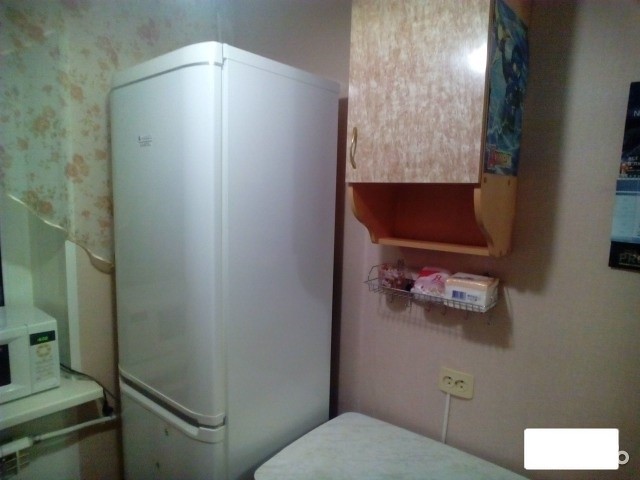In a quaint, somewhat cluttered kitchen corner, a white, apartment-sized, retro-style refrigerator with a bottom freezer stands prominently. Adjacent to it on the right, a wooden wall-mounted cabinet, adorned with a beige and rose-tinted door featuring a mottled pattern, holds a metal rack underneath, filled with various items. This cabinet also appears to have a towel or paper towel rack attached beneath it. Just barely visible atop this cabinet is a hint of a picture frame or some decorative element. 

To the left of the refrigerator, a kitchen window dressed with sheer white curtains, adorned with pale brown or yellow flowers, filters light into the space. A small microwave peeks into the frame, positioned on a counter near the refrigerator. The wall behind these elements is painted a soft, rosy pink, punctuating the cozy aesthetic of the compact kitchen scene.